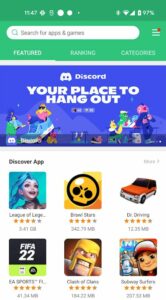This is a detailed screen capture from what appears to be a mobile device, showcasing a section of an app store interface. Dominating the top of the screen is a green header adorned with various icons and symbols. Directly beneath this is a prominent white search bar, emblazoned with text prompting users to "search for apps and games."

Following the search bar, there are navigational options in white text labeled "Featured," "Ranking," and "Categories." The primary focus just below this navigation bar is an app promotion for "Discord," highlighted by the tagline "your place to hang out" and accompanied by an array of colorful, diverse characters.

Descending further, a showcase of popular apps is displayed, featuring titles such as "League of Legends," "Brawl Stars," "Dr. Driving," "EA Sports," "Clash of Clans," and "Subway Surfers." These selections are indicative of trending games that users can download and play on various mobile devices such as iPads, iPhones, or other smartphones.

Overall, this screen capture provides a clear snapshot of a mobile app store's interface, emphasizing search functionality, navigation options, featured apps, and trending games, reflecting a user-friendly design aimed at simplifying app discovery and download.